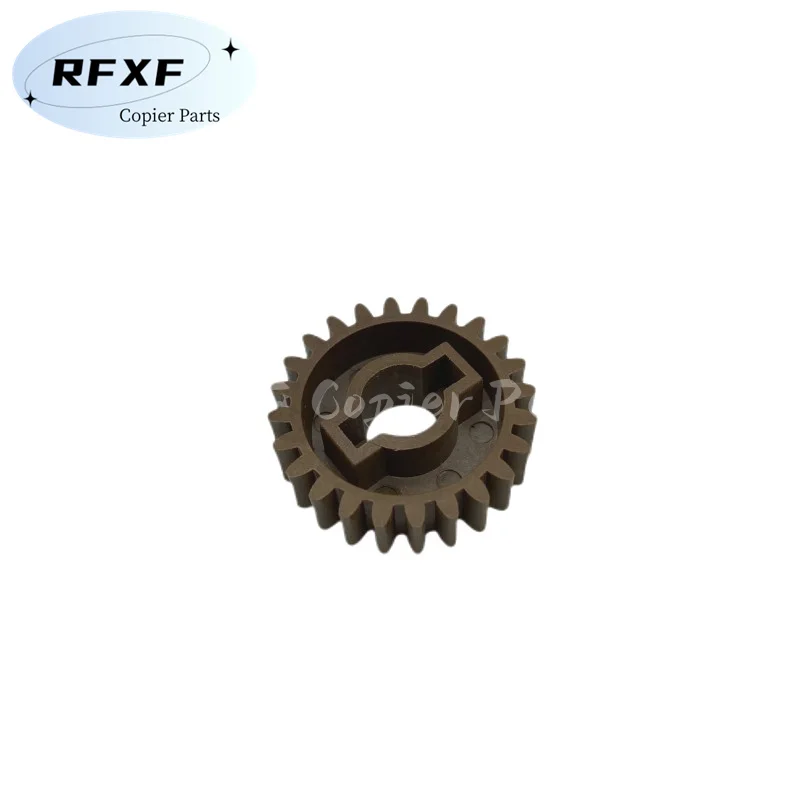The photograph captures a brown cog, positioned centrally on a flat white surface, with the overall image shape being a rectangle where the left and right sides are twice the length of the top and bottom sides. The cog, which appears to be made of formed plastic and could be 3D-printed, features multiple nubs and a central hole. In the top left corner, a blue sideways oval contains the black text "RFXF copier parts". Additionally, semi-transparent gray text reading "RFXF copier parts" overlays the center of the image.